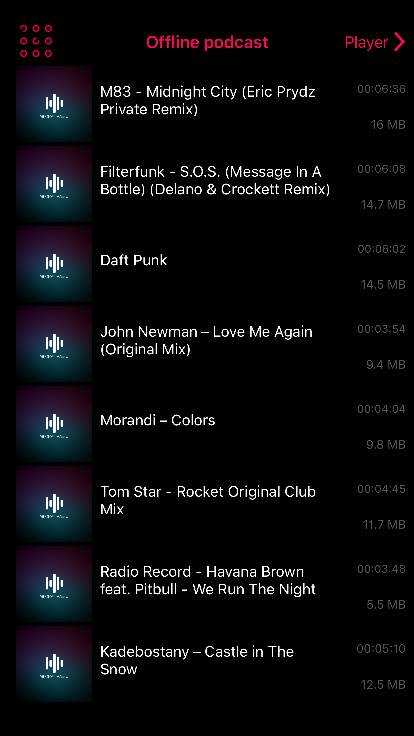The image appears to be a segment of a website, possibly optimized for viewing on a mobile phone or tablet. At the top left corner, there's a black background featuring a distinct design: a square grid consisting of three rows and three columns of red circles. Directly below this grid, the text "Offline Podcast" is prominently displayed in red, and to the right of this text, there's a playback button represented by an arrow icon.

Beneath this header, there is a list of different media entries with white sound wave icons to the left of each listing, suggesting audio content. The first entry is titled "MBS, Midnight City, E&C Fills, Private Remix." Though the fine print, which likely indicates the file size and duration, is too small to read, the list continues with:

- "Filler Funk, SOS, Message in a Bottle, Dilarbo and Crooked Remix"
- "Daft Punk, Josh Newman, Love Me Again, Original Mix"
- "Morade, Coors, Tom Star, Pockets, Original Club Mix"
- "Radio Record, Hawa, Farrah Brown featuring Peeble, We Were on the Night"
- "Katie Bustery, Castle in the Snow"

Despite the 'Offline Podcast' branding, these listings seem to be song titles or music remixes rather than traditional podcast episodes.